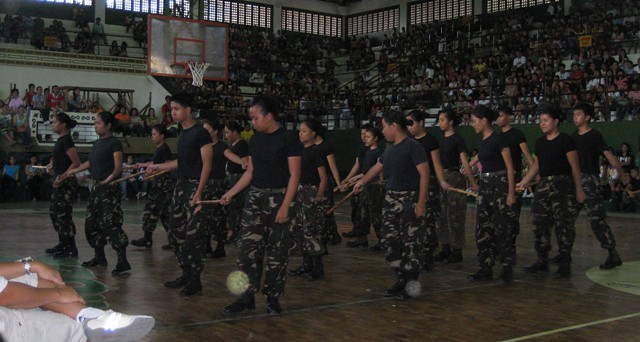In this photograph, taken inside a gymnasium or basketball court, multiple people are engaged in what appears to be a highly coordinated dance routine or military drill. The gym features a clear acrylic backboard with orange edging, an orange metal rim with a white net, and brown wooden flooring marked with various white and gray basketball court lines. Along the walls, there are several rows of bleachers populated by audience members watching the spectacle. In the center of the court, numerous participants, both male and female, are dressed in black short-sleeved t-shirts and camouflage pants. Each person is holding a wooden stick, which they move in sync as part of their choreographed movements. Some small balls are visible, bouncing on the ground, suggesting an element of complex coordination. The setting also includes a man seated in the bottom left corner of the image, cross-legged with his hands on his knees, overseeing or perhaps participating in the activity. The scene is bustling with energy, indicative of a halftime performance, a special drill routine, or a dance performance designed to entertain the crowd.